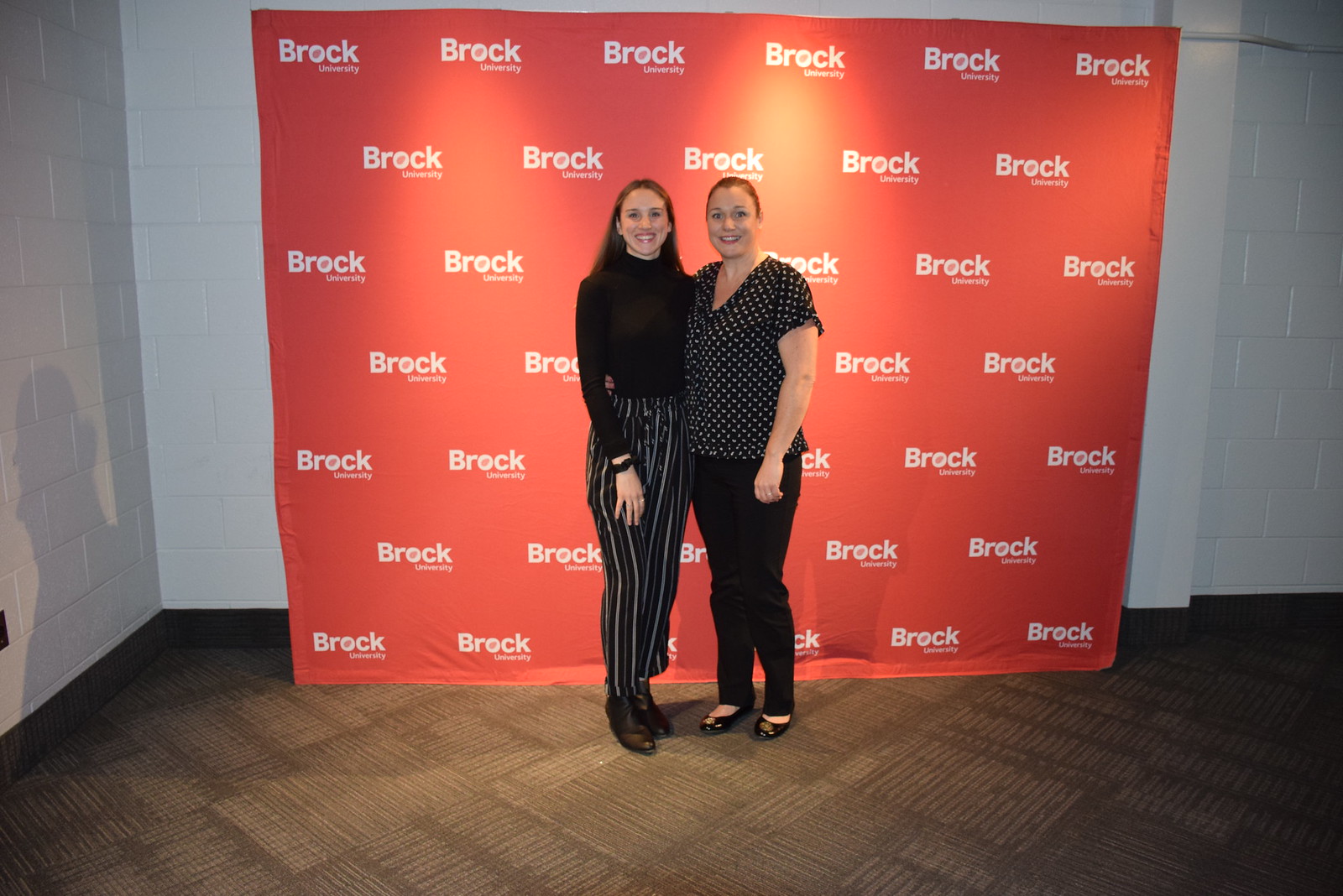This photograph captures two young women standing arm in arm, beaming with joy. Both are white, with the one on the left sporting long brown hair, a black turtleneck, black and white striped pants, and black boots. The woman on the right has brown hair pulled back in a ponytail, wearing a black and white polka-dot blouse with a v-neck, black pants, and black shoes. They are positioned against a large red backdrop emblazoned with the words "Brock University" in white letters. The backdrop is set in front of a white cement wall, and they are standing on a brown carpeted floor. The atmosphere is warm and cheerful, capturing a moment of happiness and camaraderie.